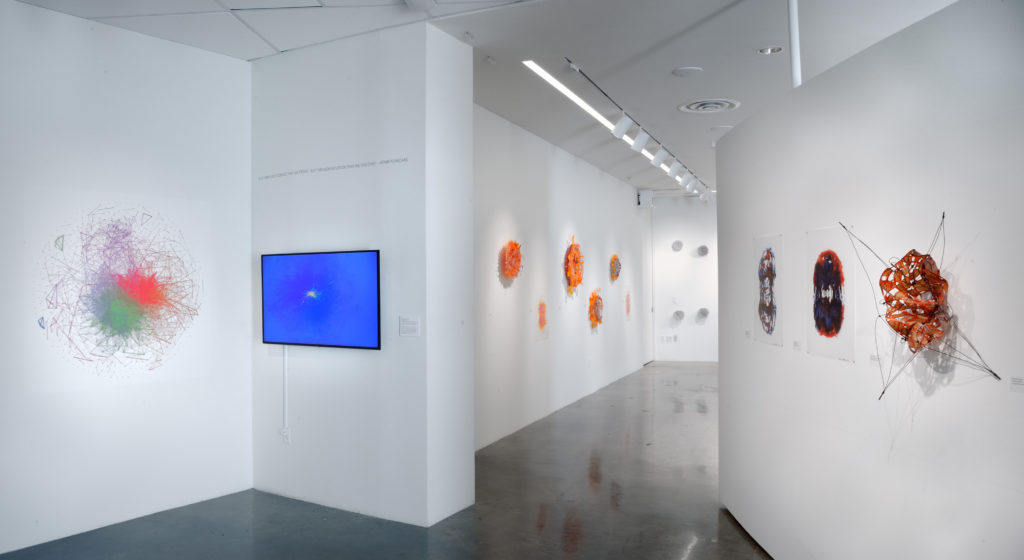The photograph captures a modern art museum with pristine white walls and a sleek, shiny gray marble floor. Illuminated by fluorescent white lights from above, the space exudes a contemporary feel. On the left wall closest to the viewer is a striking painting of a brown orchid flower, with a protruding pistil and an adjacent elaborate wire four-point star. Moving further down the wall, one encounters what seems like a chaotic splash of red and green paint with scattered lines, almost resembling a cloud of colors. Adjacent to this is a flat screen TV with a blue display and a white crack through the center, adding a digital element to the traditional gallery setup. On the right wall, a collection of vibrant art pieces includes balled-up wires in a variety of colors—orange, green, and purple. One piece, in particular, resembles a gigantic, glazed walnut. Towards the end of the left wall, a series of orange wreaths adds a cohesive element with bursts of color. The overall scene is one of eclectic modern art, devoid of any anthropomorphic designs, emphasizing abstract and unconventional forms.